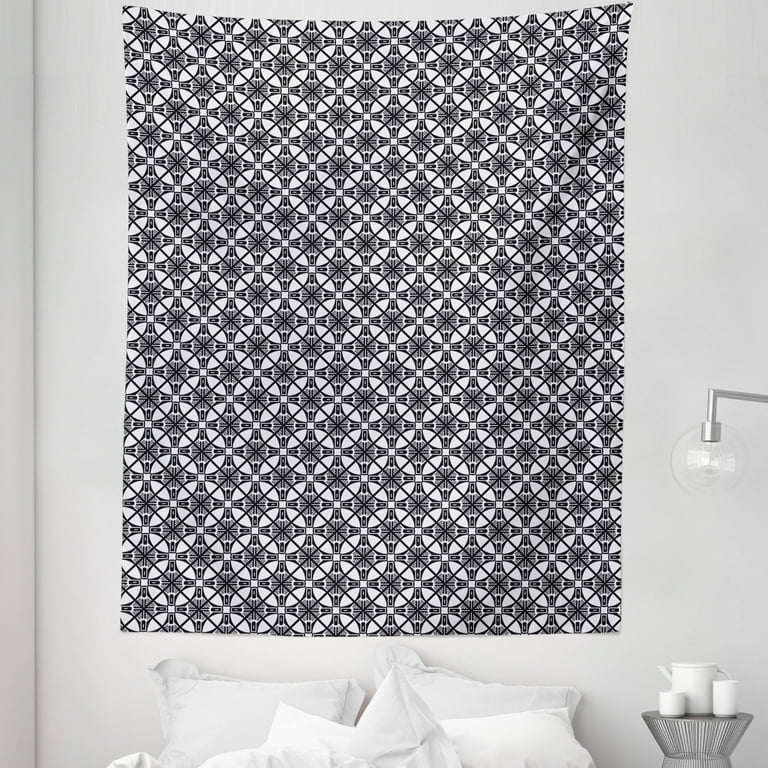In this bedroom, a white wall serves as the backdrop for a pinned-up tapestry adorned with a repetitive pattern of black diagonal lines intersecting with white circles, creating an intricate geometric design. Below the tapestry, a bed is partially visible, characterized by an assortment of four to five white pillows, some with ruffled edges, set against white bedding. To the bottom right of the image, there is a stylish stand or small table. On this table, three white mugs and a smaller teacup are neatly arranged beside a framed picture. Also on the right side of the image, a floor lamp with a silver metal frame and a clear glass globe adds a touch of modern elegance to the room's interior decor.